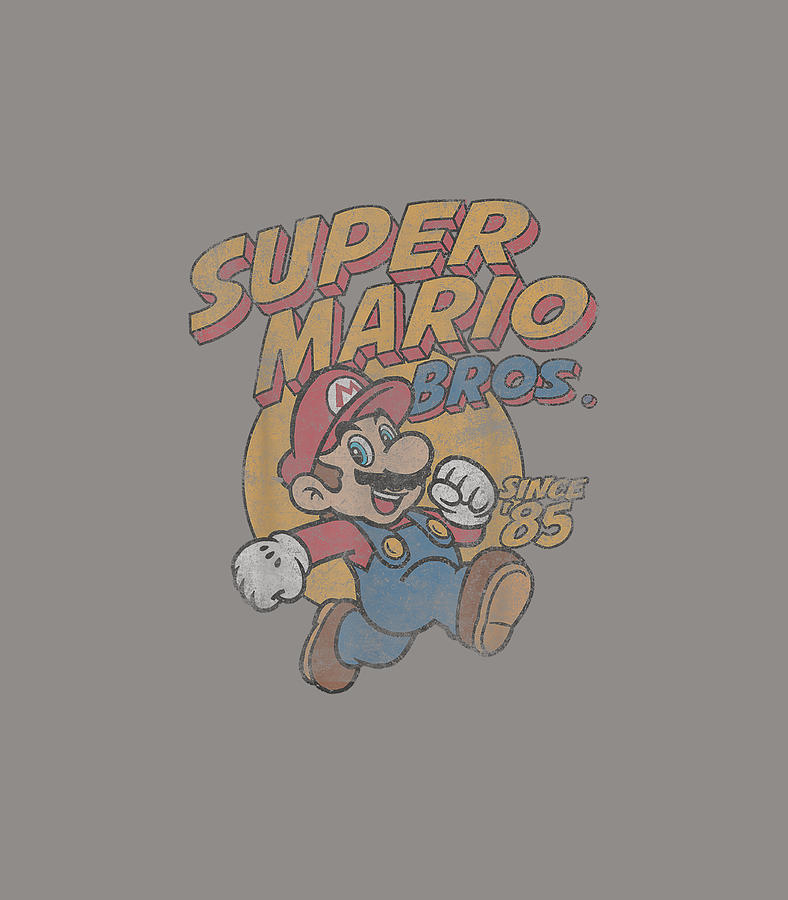The image depicts a vintage logo of the iconic Super Mario Bros game by Nintendo. Centrally featured is Mario, the beloved character, characterized by his distinct appearance: a black mustache, blue eyes, and a red cap with the letter 'M' prominently displayed. He is dressed in his classic blue overalls, a red long-sleeved shirt, white gloves, and brown shoes. Mario strikes a running pose, with his legs and arms positioned in a dynamic movement, suggesting action. He is set against a yellow circle resembling a sun, placed on a gray background. Above Mario, the text "Super Mario Bros" appears in a 3D font style, with "Super Mario" in yellow lettering shaded in red and "Bros" in blue lettering shaded in red. Below him, the caption reads "Since '85," indicating the game's release year, written in yellow. The vintage graphic appears slightly faded and blurry, enhancing its retro charm.